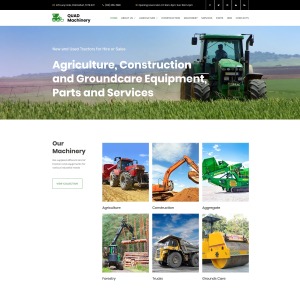In the foreground, a green tractor with large wheels dominates the scene. To the right of the tractor, a black bar with text, albeit partially blurry, appears to contain the word "machinery." The background is a blend of blue hues and agricultural fields with grass, with scattered buildings and distant hills completing the horizon. Above the main image, a distinct black bar stretches across, adding contrast. The entire composition appears as a collage of six distinct images, each depicting various aspects of agricultural and construction machinery. These include a red tractor, blue dirt, construction scenes, trucks, and a particular instance of gray machinery set against a snowy backdrop, featuring a gray roller and green trays at the rear. The overall theme revolves around agricultural equipment and machinery in diverse environments.